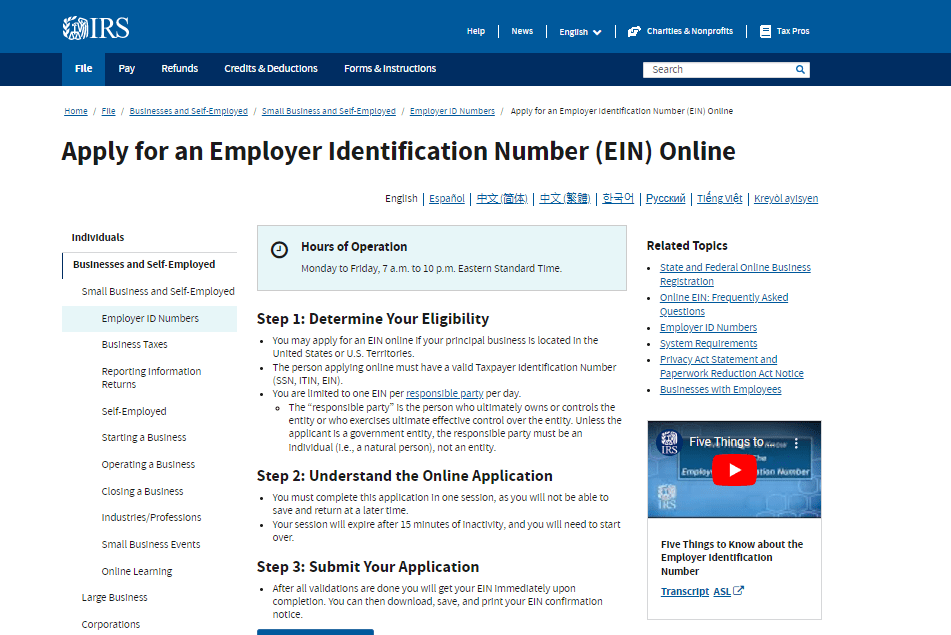This image displays a webpage from the official IRS site. At the top, a prominent blue header features the IRS logo and the acronym "IRS." On the right side of this header, there are several options such as "Help," "News," and "English," each separated by vertical lines. There is also a dropdown arrow next to the language selection.

Below the header, the first major section is geared towards non-profits and tax professionals, indicated by corresponding subheadings like "Home" and "Apply for an Employer Identification Number (EIN)," with "EIN" in parentheses. This section also features subheadings in various languages including English, Spanish, and an Asian script, accommodating a diverse audience.

Highlighted within a light blue rectangle are the hours of operation: Monday through Friday, 7 AM to 10 PM Eastern Standard Time.

The webpage is structured into three main steps for applying for an Employer Identification Number (EIN):

1. **Determine Your Eligibility**: Contains three bulleted points outlining specific criteria.
2. **Understand the Online Application**: Provides detailed bulleted instructions on the application process.
3. **Submit Your Application**: Concludes with essential steps for completing the application, accompanied by bulleted information.

Towards the bottom, there is a section titled "Related Topics" featuring bulleted links for additional resources, and a media element with an image of a video, potentially serving as a tutorial or informational guide.